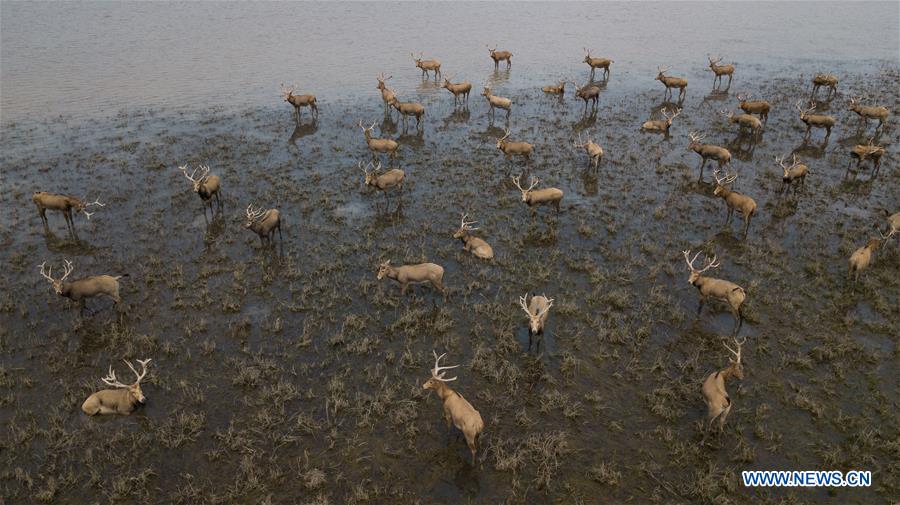This image shows a large herd of elk in a wetland area, characterized by a mix of water and grassy patches, stretching across the entire frame. The elk, predominantly brown in color, are distinguished by their large, majestic antlers, though a few antlerless females are also present. They occupy various positions, with many standing and a few resting on the muddy terrain. The background hints at water meeting the ground, creating a rich, soggy environment typical of wetlands. This diverse assembly of elk evokes a sense of tranquility and natural beauty amidst the marshy landscape.